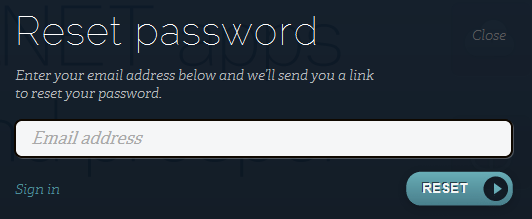The image appears to be a screenshot of a website, showcasing a "Reset Password" page against a navy blue background. The word "NET" is prominently displayed in all caps, subtly darker than the background, while "apps" is written in lowercase, all in the same blue hue.

At the top of the screenshot, there is a white, thin font that reads "Reset Password," and on the far right, the word "close" is displayed in a light gray color. 

Below the "Reset Password" heading, the instructions are given in a smaller white font: "Enter your email address below, and we'll send you a link to reset your password."

A text input box spans nearly the full width, featuring a faded placeholder text “email address.” Below this input field, to the left, is a blue-colored link that says "Sign in." On the far right, there is a baby blue, pill-shaped button with the word "Reset" written in white. Next to the "Reset" button, there is a small black circle containing a right-pointing baby blue triangle, resembling a play button.